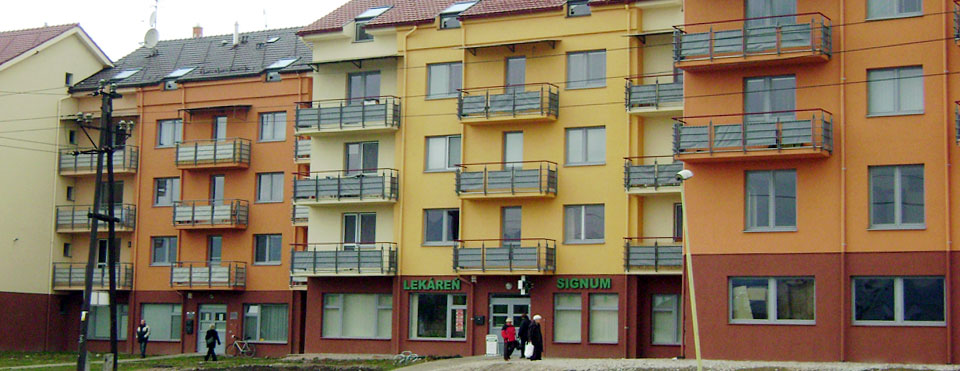The image depicts a row of four connected apartment buildings, each spanning four stories. The top three floors feature balconies with sliding glass doors, while the ground floor houses storefronts. The buildings are painted in a variety of muted tones—light beige, orange, cream, and yellow. In particular, the yellow building has a storefront labeled "LeCarin Signum," suggesting a European style pharmacy with the characteristic green cross sign. The balconies span across different vibrant shades, complementing shingled roofs in red and black. To the far left, an additional tall building with off-white walls and a red roof stands adjacent to the row, potentially another apartment but with a distinct house-like silhouette. Scattered in front of the buildings are about five people, some gathered near the storefronts, adding a touch of daily life to the scene.